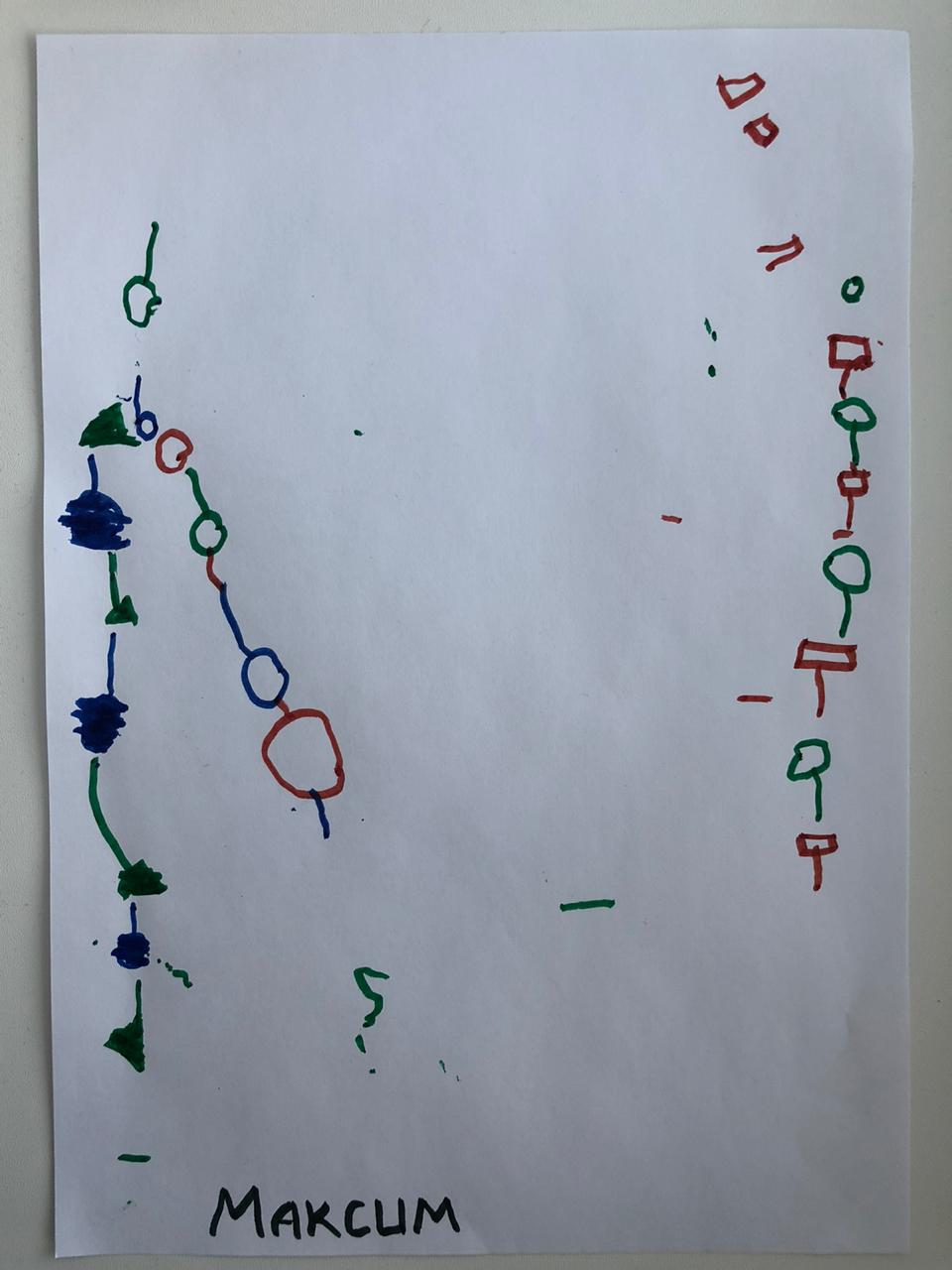The image showcases a photograph of a piece of paper adorned with various colored markings. The paper is set against a cream-colored background, which could be either a table or a wall, as the exact surface is ambiguous. The photograph is captured in portrait orientation. 

Starting from the bottom left corner, there is a dark blue inscription that reads "M-A-K-C-U-M." Above this, several distinct shapes and colors form a complex pattern. There is an alternating sequence of blue and green elements: a green shape with an upward line, followed by a blue streak with lines pointing up and a slight rightward curve. This pattern continues with another blue streak featuring a wavy green line, followed by a blue shape with an upward blue line. 

Also present is a green triangle with an upward green streak, and a large blue blob with a vertical line. Further up, a green triangle and a blue circle that resembles the letter 'B' are seen. Above this 'B' shape, there is a green circle with an upward protruding line. 

Intersecting this point, a red circle is connected through a series of lines going downward: a green one leading to another green circle, a red line to a blue circle, a red line to a red circle, and a blue line leading to another blue circle. 

On the right side, a mirror-like pattern exists, featuring alternating red rectangles and circles with lines stretching downward. This sequence continues with red rectangles and green circles, leading up to the upper right corner of the paper. The intricate design exhibits a lively interplay of colors and shapes, creating a visually striking composition.